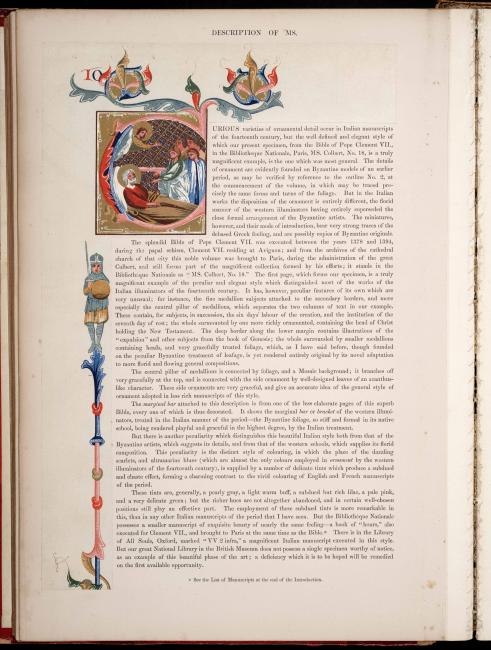This color photograph, taken in portrait orientation, captures a detailed view of an open, aged illuminated manuscript. The left page is fully visible, while only part of the right page is seen. The book's binding is noticeably coming apart, suggesting its vintage nature. At the top left of the page, a richly colored Renaissance-style illustration depicts a person lying in bed, surrounded by doctors and several angels behind the figure. Above this scene, ornate decorations featuring red, blue, and cream colors frame the text "Descriptions of," though the rest is obscured by artifacting. Below, a vertical illustration shows a soldier atop a segmented pole with ball finials, brandishing a sword and shield in red, blue, and flesh tones. The remaining page is filled with paragraphs of black text in a foreign language. The manuscript combines realistic artistic elements with historical visual themes, echoing the style of Victorian-era and religious paintings.